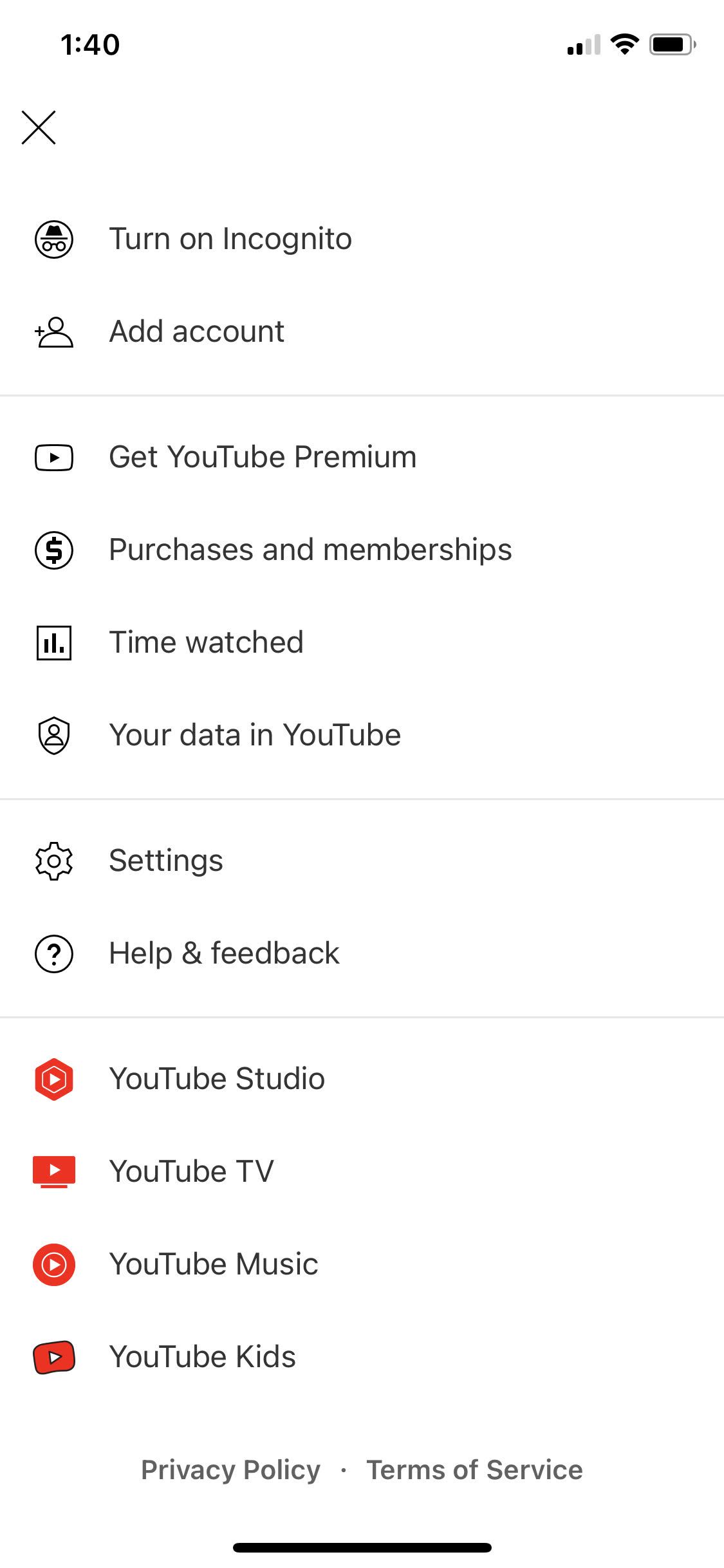The image displayed on a cell phone screen features a nearly fully charged battery icon and a strong connection indicated by two signal bars. The time is shown as 1:40, with an 'X' icon directly below the time. 

The screen is divided into several sections with different options, each accompanied by an icon to the left of the option description. The sections are as follows:

1. **Incognito and Account Management**:
   - **Turn on Incognito**
   - **Add Account**

2. **YouTube Services and Data**:
   - **Get YouTube Premium**
   - **Purchases and Memberships**
   - **Time Watched**
   - **Your Data in YouTube**

3. **Support and Settings**:
   - **Settings**
   - **Help and Feedback**

4. **YouTube Platforms**:
   - **YouTube Studio**
   - **YouTube TV**
   - **YouTube Music**
   - **YouTube Kids**

Each YouTube-related option is represented by a red icon similar to the standard YouTube symbol. At the bottom of the screen, there is some smaller text reading "Privacy Policy" followed by a small dot, and "Terms of Service." Below this text, there is a thin black bar extending horizontally from left to right across the screen. 

There is no additional text or imagery on the screen.